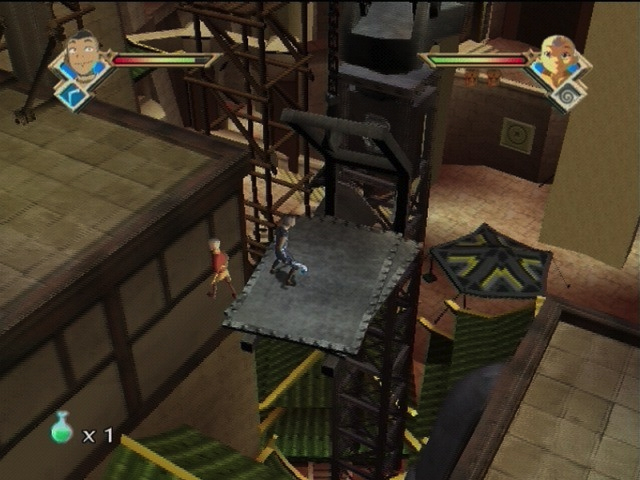This image is a screen capture from a cartoon-styled video game. On the left and bottom right of the screen, there are structures with beige tiled roofs and wooden outlines. At the center is a tall metal lattice tower featuring an outward-pointing platform towards the viewer. Below the platform, traditional East Asian-style roofs, adorned in green with gold outlines, add a cultural touch to the setting.

Standing on the metal platform are two distinct characters. On the left, a character wearing an orange top, yellow bottom, and brown shoes is precariously hanging off the edge, yet still level with the platform. This character is bald and seems to be in a perilous position. On the right, standing firmly on the platform, is a character dressed in all blue with short sleeves. He wields a bright blue boomerang and has a mostly shaved head, leaving just a small amount of hair on top.

Additionally, there are status icons for each character: On the left side of the screen, an icon depicts the half-shaven character with a health bar extending to the right, colored red to green. On the right side, the bald character in yellow has a health bar extending to the left, similarly colored red to green, accompanied by a blue arrow.